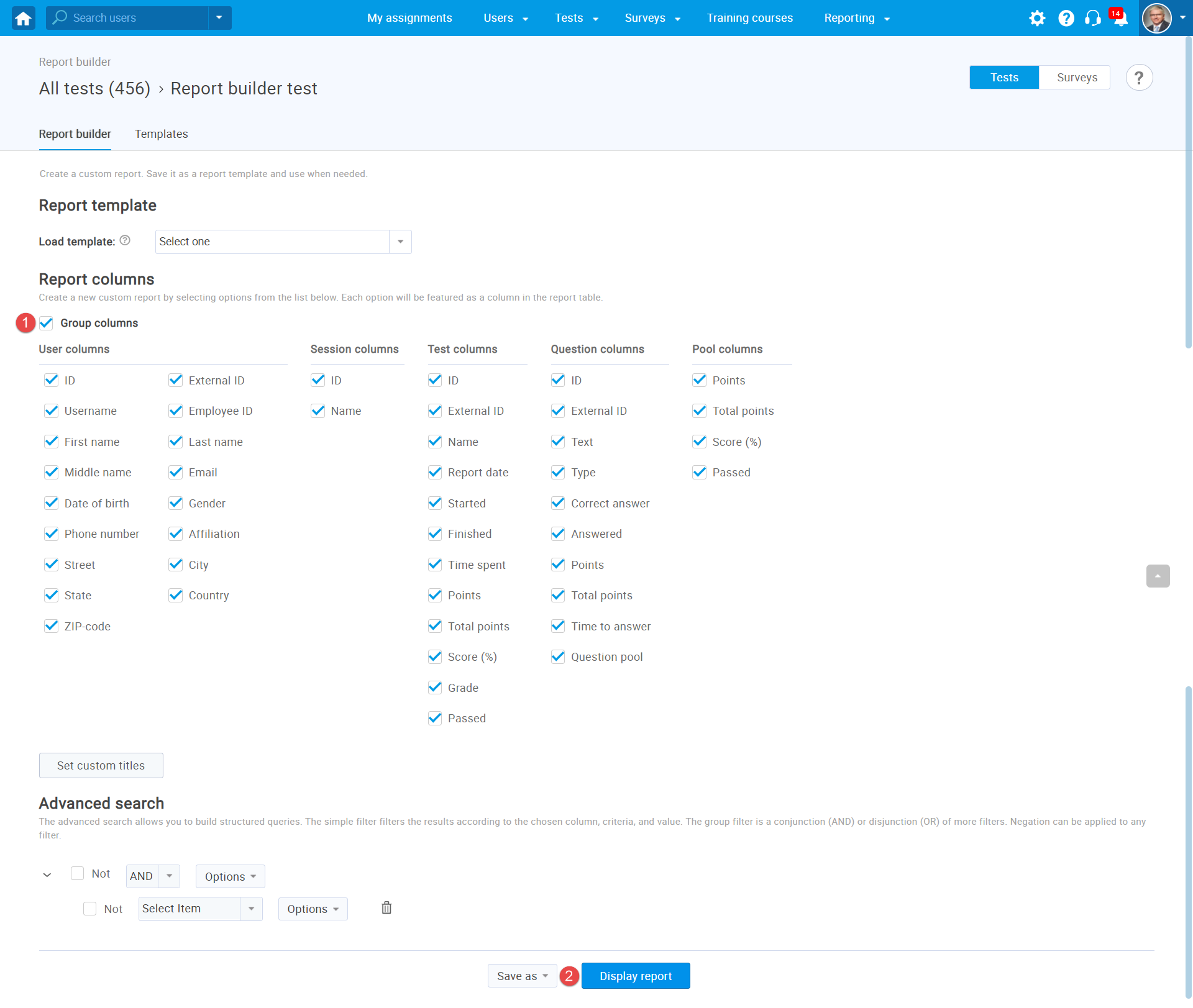The image appears to be a screenshot from a website, specifically an interface related to report building. At the top, the header consists of a light blue rectangular banner with clickable white text links. The navigation options available include "My Assignments," "Users," "Tests," "Surveys," "Training Courses," and "Reporting."

To the right of these navigation links, there are several icons, including a bell icon displaying the number 14, which likely indicates the number of notifications, and a square icon for messages. Alongside these, there's a small profile picture of a man with blonde hair, wearing a suit and tie, and black glasses.

Beneath the header, the upper section of the interface continues with a faint blue background. This area indicates headings such as "Report Builder," "All Tests (456)," and "Report Builder Test." Below this, there is an instructional segment labeled "Report Builder" with additional text stating, "Templates: Create a custom report, save it as a report template, and use when needed."

Further down, there is a section for loading templates, with a dropdown menu labeled "Select One." Finally, at the bottom of the image, in the "Report Columns" area, there are multiple checkboxes, all marked as checked, indicating that every column option has been selected. The background of this lower section is entirely white.